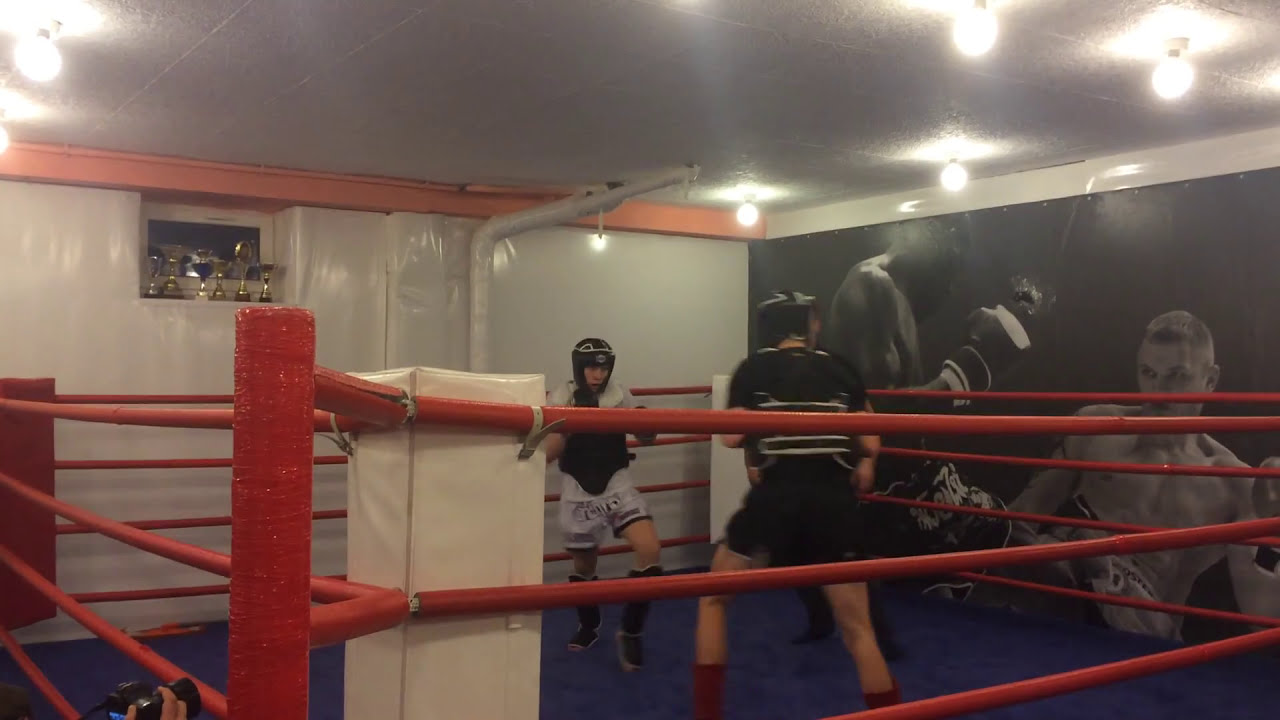This photograph captures an intense moment inside a cramped boxing ring where two men are sparring. Both boxers are in full gear, including black and white headgear and helmets. One fighter wears a black outfit with white stripes and red socks, while the other sports a white outfit with black and red accents paired with dark socks. The boxing ring features red ropes, white and red corners, and a blue mat. The background reveals gray and white walls with orange and white trim, a poster on the right depicting two men fighting, and a window on the top left adorned with several trophies. The gym itself has a low ceiling with bright lights illuminating the scene. The focus of the image is squarely on the two fighters at the center of the ring, with no coaches or other students visible.